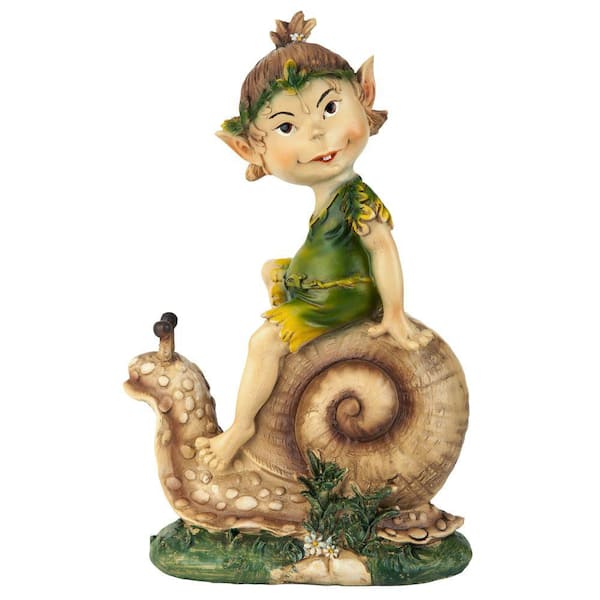This photograph showcases a whimsical garden statue of a fairy-like elf girl seated on a large snail, set against a white background. The elf girl has an impish smile, exposing her two prominent front teeth that resemble little buck teeth. Her hair is styled in a high ponytail, partially covered by a green leafy headband or crown, with some of her green-tinted hair peeking through. She features striking pointed ears and almond-shaped eyes, exuding a cherub-like charm. Dressed in a short, Peter Pan-inspired green and yellow outfit accented with leaf motifs, she sits with her bare legs visible from the knee down. One leg is draped over the snail’s neck while the other is obscured from view. Her left arm rests on the snail’s back, thumb pointing forward. The large, brown snail, detailed with dark spotting and extended eyestalks, sits in a patch of green grass interspersed with flowers and tiny bushes. This detailed resin or acrylic figurine captures a playful and magical essence, inviting viewers to imagine a miniature, enchanted world.